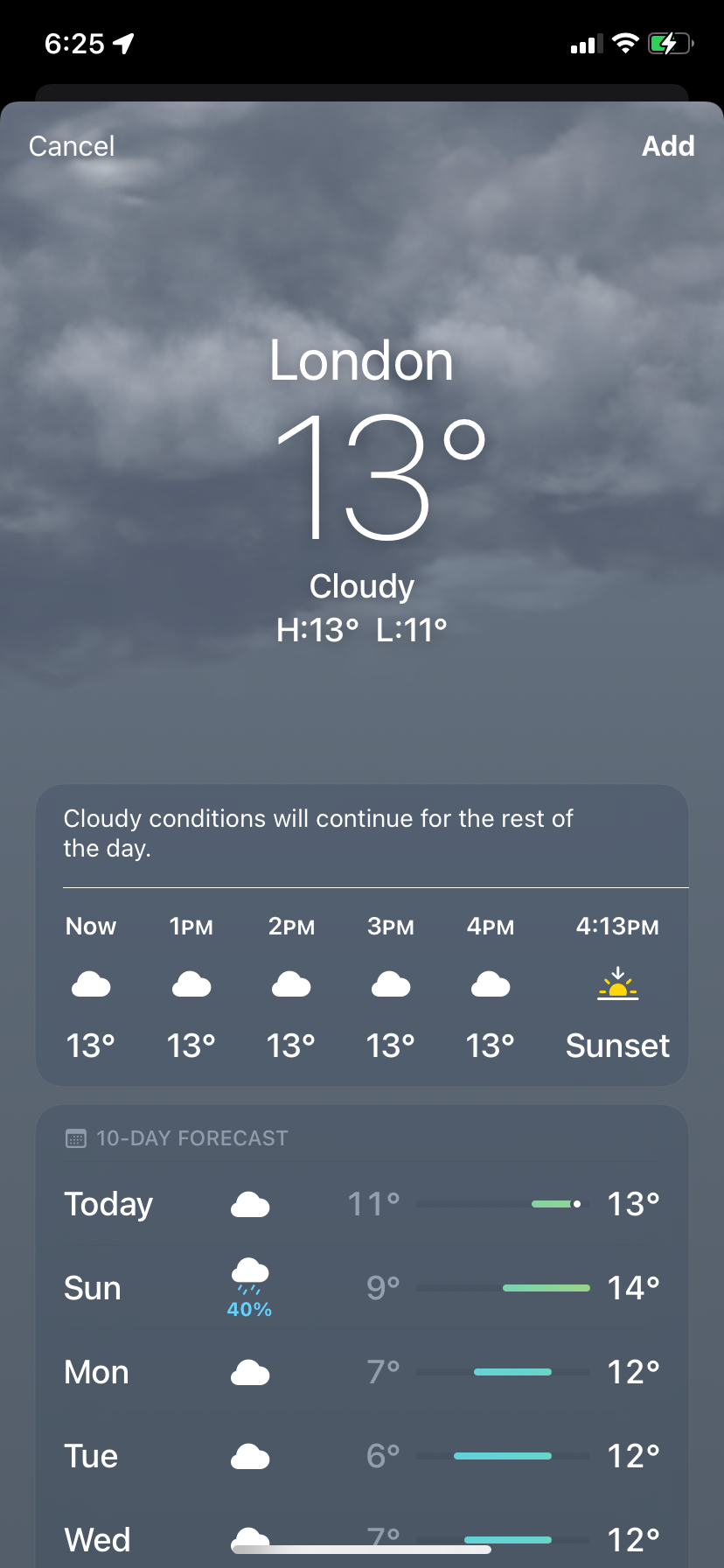The screenshot captures a smartphone display showcasing weather information. At the very top, a black banner displays "6:25" in white text. To the right of the time, icons for Wi-Fi signal, cell signal, and a battery with a lightning bolt symbol indicate the phone is charging.

Below the banner, the weather section is presented with a mostly gray and white cloudy background. At the top left, the word "Cancel" is written with a capital "C," and on the right, "Add" is also capitalized. 

The primary weather information indicates that it's for London, with "London" written with a capital "L." Underneath, the temperature is displayed as "13°," accompanied by text stating, "Cloudy. High: 13°, Low: 11°." A brief forecast mentions, "Cloudy conditions will continue for the rest of the day."

A timeline showing the weather for specific hours follows, listing "Now," "1 PM," "2 PM," "3 PM," and "4 PM." "4:13 PM" is highlighted as the sunset time.

Further down, a "10-day forecast" section begins with the days of the week: "Today," "Sunday," "Monday," "Tuesday," and "Wednesday." Icons and percentages detail the weather predictions, such as a cloud icon with "40%" indicating a chance of rain. Temperature predictions for the forthcoming days are listed as "11°," "9°," "7°," "6°," and "7°," respectively.